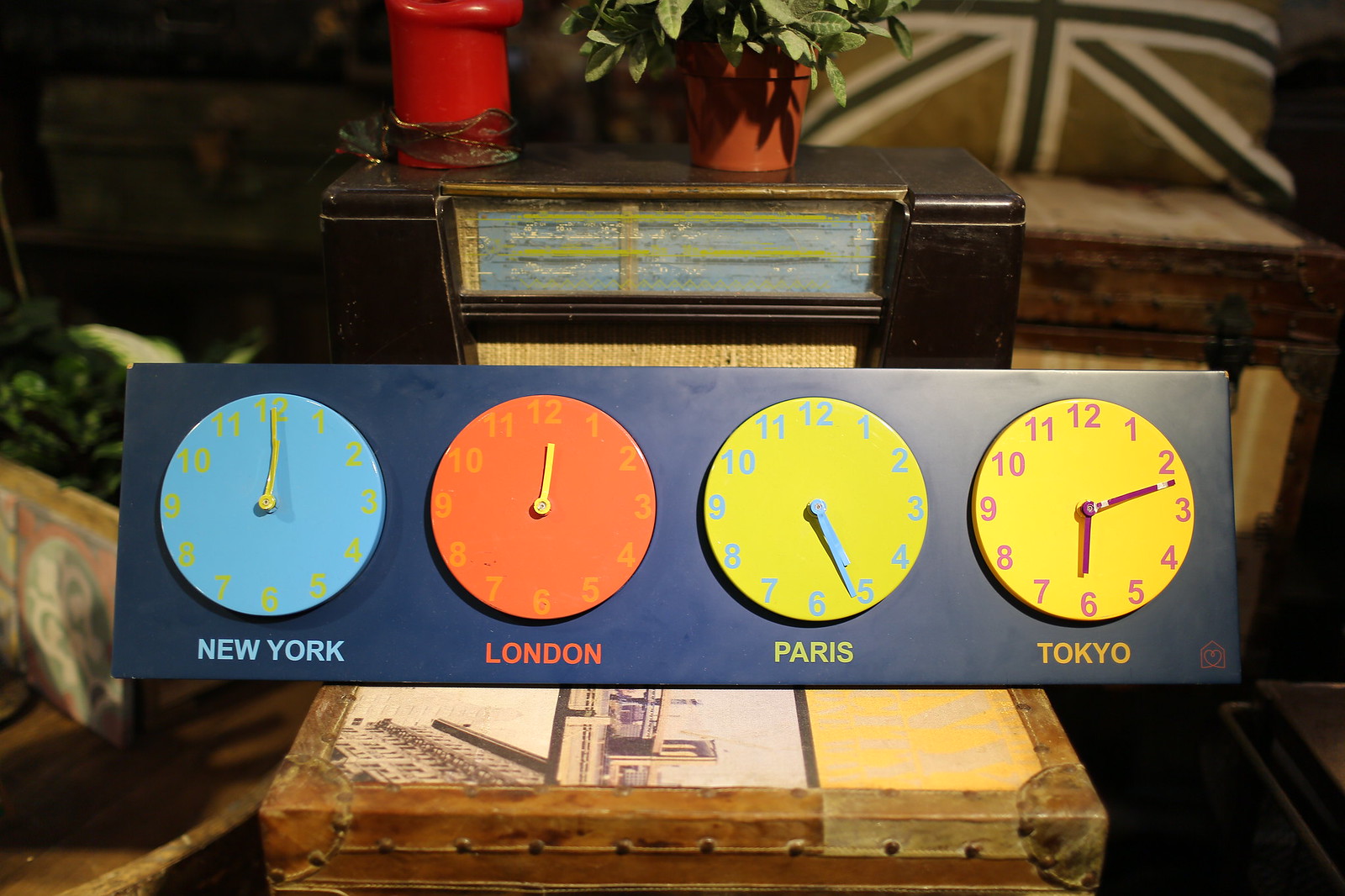In this image, we see a wooden plaque with four manually set clocks mounted on it, each painted in a different color to represent various cities around the world. The plaque is blue and gives a bit of a playful or vintage feel. 

1. The first clock on the left is a blue round clock designated for New York, and it shows 12:00.
2. Next to it, the red round clock represents London, also indicating the time as 12:00.
3. The third clock, a yellow round one, denotes the time in Paris, set to approximately 5:26.
4. The clock on the far right is another yellow round clock with red numbers, representing Tokyo, showing the time as 6:12.

All these clocks are placed on an antique-looking box, contributing to the overall charm. In the room's background, there is a cozy couch adorned with pillows, a plant, and an antique radio on the coffee table. The scene suggests a blend of modern living with nostalgic elements, creating a warm and inviting atmosphere.